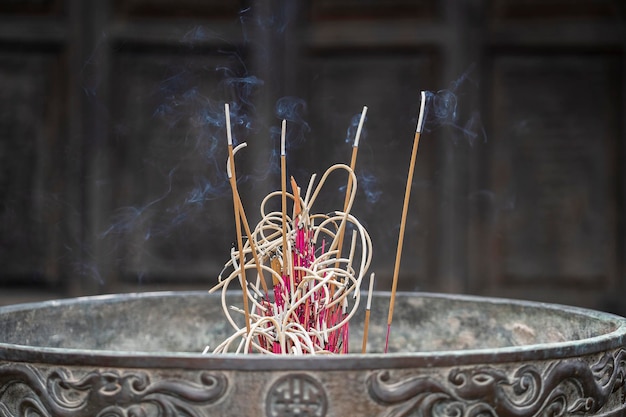This close-up image captures a detailed scene of burning incense sticks in a large, cylindrical bowl. The bowl appears to be made of a stone or metal material with a grayish-bronze, silvery color and intricate carvings, possibly depicting animals or dragons. The edges of the bowl can be seen at the bottom of the photograph. Inside, the bowl holds five upright incense sticks, primarily brown with white tips where ash has formed, and white smoke gently wafting from them. In the midst of these sticks, a bundle of intertwining red and white elements forms a central ball, mingling with the smoke from the burning incense. The background is dark and blurry, hinting at a dark brown or black wall or door, with a slight purple tinge, creating a stark contrast that emphasizes the intricate and meditative focus of the incense scene in the foreground.